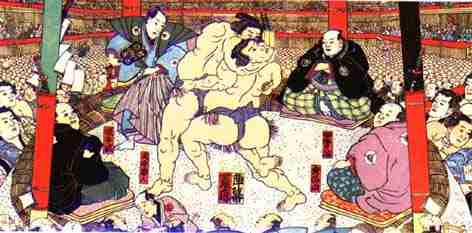This is a detailed illustration depicting a sumo wrestling match. Two very large, heavyset sumo wrestlers, dressed in traditional loincloths, are intensely grappling; one wrestler has the other in a neck hold while the other attempts to push him off or grab him for a throw. Four individuals, dressed in traditional Japanese robes, are seated almost directly on the stage, closely watching the match; one of them, in a black robe, may be a judge or an important person in the scene. Surrounding this intimate ring-side group is a vast crowd of spectators, all attentively watching the intense competition. The composition is primarily in muted tones with accents of reds and blacks, suggesting an older, perhaps historical, setting. The characters in the background are rendered small, emphasizing the focus on the wrestlers and the immediate spectators. Overall, this richly detailed and vividly colored artwork captures the intensity and tradition of a sumo wrestling event.